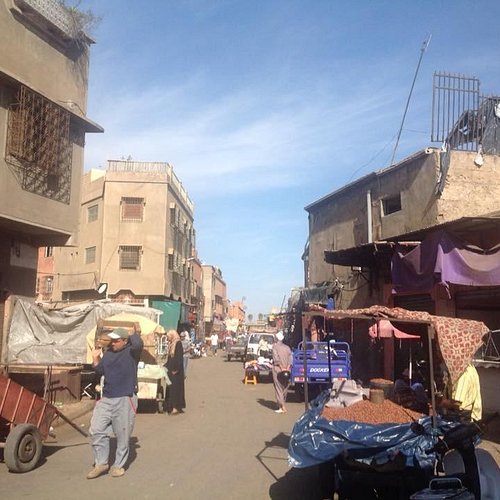This photograph, taken during the daytime, depicts a bustling street scene, likely in a Middle Eastern or third-world country. The sky is a bright blue with minimal cloud coverage, enhancing the vivid contrast with the earthy tones below. The street itself is unpaved, composed of brown dirt, and is flanked by buildings that appear to be made of clay or sheetrock, characterized by their flat, boxy shapes and numerous windows—some with bars for security.

On the left side of the image, there are multiple compact houses with bars on their windows, indicating a focus on safety. Similarly structured buildings are visible on the right, including one with an open window frame vulnerable to the elements. The street is filled with various vehicles, including buggies, wagons with tarps, and an older blue truck, all seemingly engaged in transporting goods.

The road is congested not just with vehicles but also with people. A man in a long-sleeve shirt is seen carrying a box over his head, potentially making a delivery. Shadows cast by the people and vehicles suggest a sunlit day. In the bottom right-hand corner, a vendor appears to be selling peanuts or similar goods, adding to the lively atmosphere of this busy street scene.